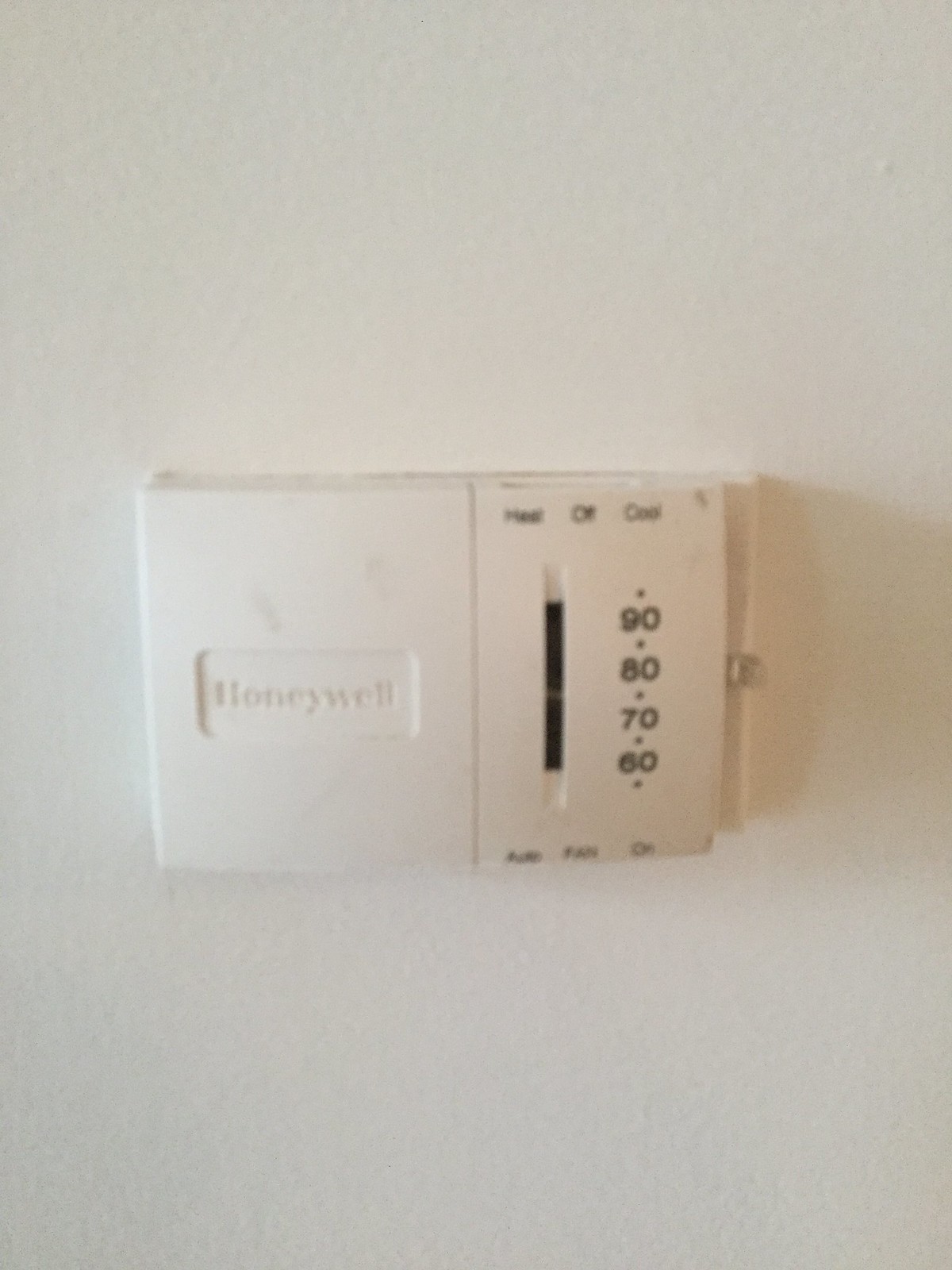This detailed color photograph prominently features a white Honeywell thermostat, centrally mounted on a pristine white wall. Positioned to the left of the thermostat's front panel is the clearly visible Honeywell brand name, spelled out in uppercase letters as "H-O-N-E-Y-W-E-L-L." To the right, the thermostat displays various command settings at the top: "Heat," "Off," and "Cool." Adjacent to these settings is a black vertical bar, clearly marked with temperature gradations of 90, 80, 70, and 60 degrees. Below this bar, the control options "Auto," "Fan," and "On" are specified.

A small, transparent lever to the right of the thermostat is designed for manual adjustment and catches the ambient light, creating a subtle reflection on the wall. The entire thermostat also casts a shadow behind it, contributing to the photograph's dimensionality. The image is oriented vertically, emphasizing the height over its width, and showcasing a clean and minimalistic aesthetic with no people, animals, plants, flowers, trees, buildings, signs, motorized vehicles, or water present in the frame.